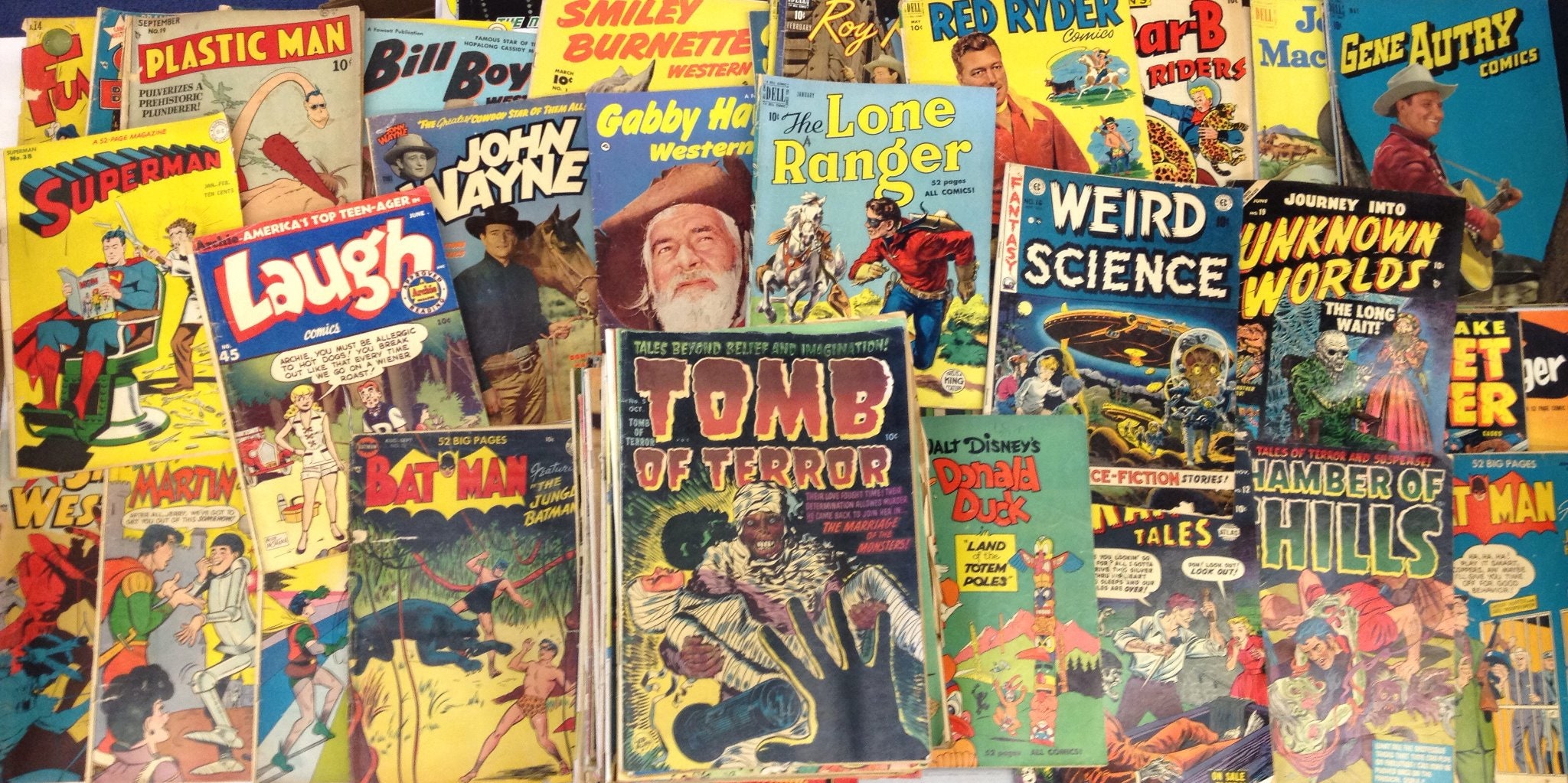The image captures a vibrant and chaotic assortment of vintage comic books and magazines scattered across a background, predominantly showcasing covers from the 1950s to the 1970s. In the front row, notable titles include a Batman comic depicting a figure in the jungle being attacked by a black panther, a Tomb of Terror comic with a black hand reaching towards a black character, and Walt Disney's Donald Duck featuring a totem pole made of ducks. Positioned above the Tomb of Terror, The Lone Ranger comic displays a white horse and the titular character in a red shirt and blue pants. To its right, a Weird Science comic features a spaceship beneath its title in white lettering. The collection also includes well-known titles such as Superman, Plastic Man, Laugh, Red Rider, Unknown Worlds, and Chambers of the Hills. The covers predominantly feature hand-drawn artwork in bright, eye-catching colors like yellow, blue, red, and green, exuding a distinctly vintage aura.